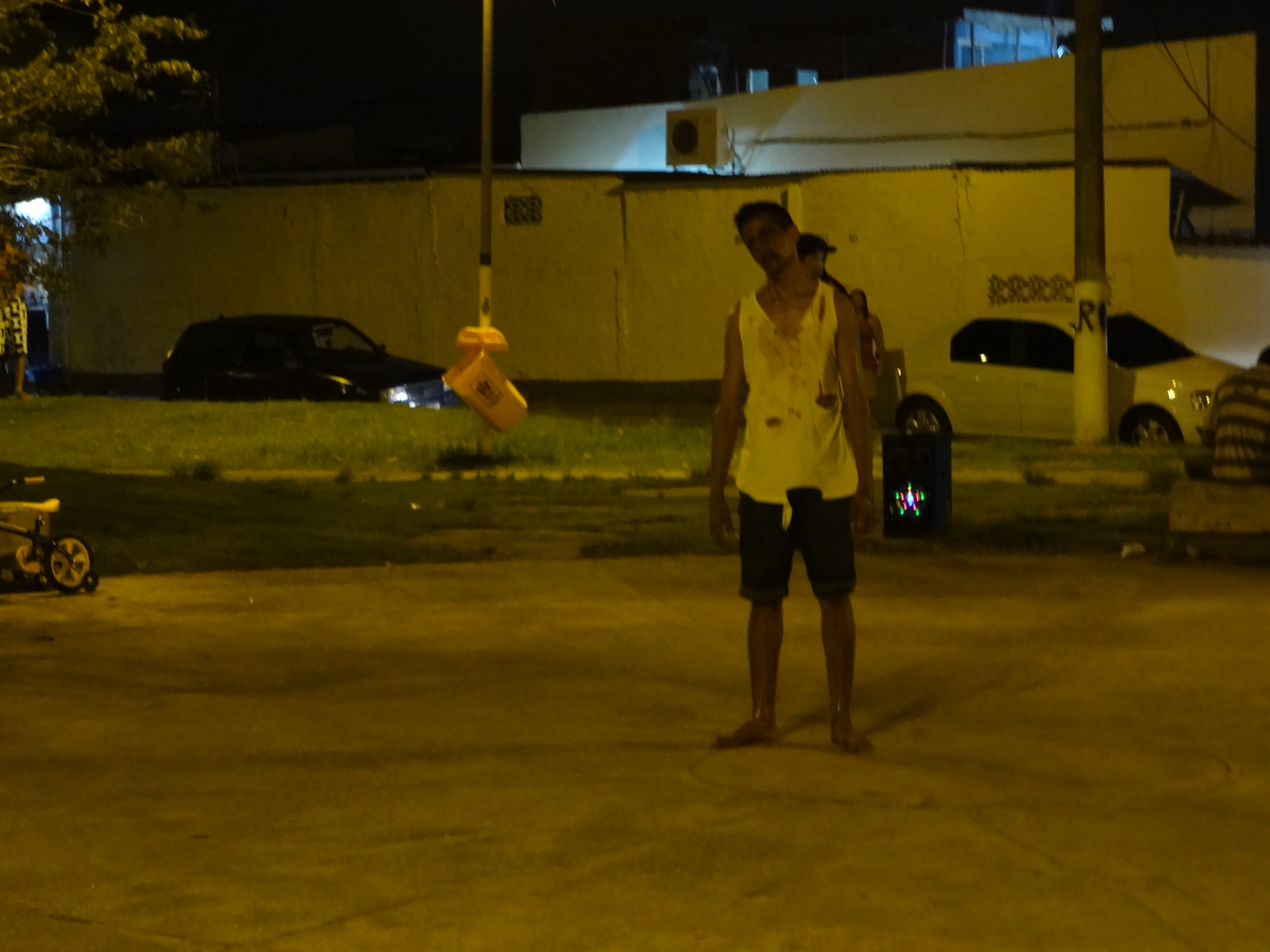In a blurry nighttime photograph, a dark-skinned man stands barefoot on a dirty, hard-packed surface, surrounded by an open area. He wears a torn, dirty, and possibly blood-stained sleeveless white shirt and black shorts that reach his knees. His head tilts slightly to the side, suggesting distress or fatigue. To his right, a white car is parked, with an upright post and a yellow trash can visible in the grassy area nearby. A black SUV is on his left. Behind him, two people are partially visible. Additionally, there is a faint outline of a striped-shirted man sitting on a bench near the white car and what looks like a child's bicycle and some kind of electrical equipment. The background includes a couple of gray walls with an air-conditioning unit and bright lights from a small black box. Despite the dim and poorly lit conditions, the scene hints at a neighborhood or park setting with a mix of human activity and urban elements.